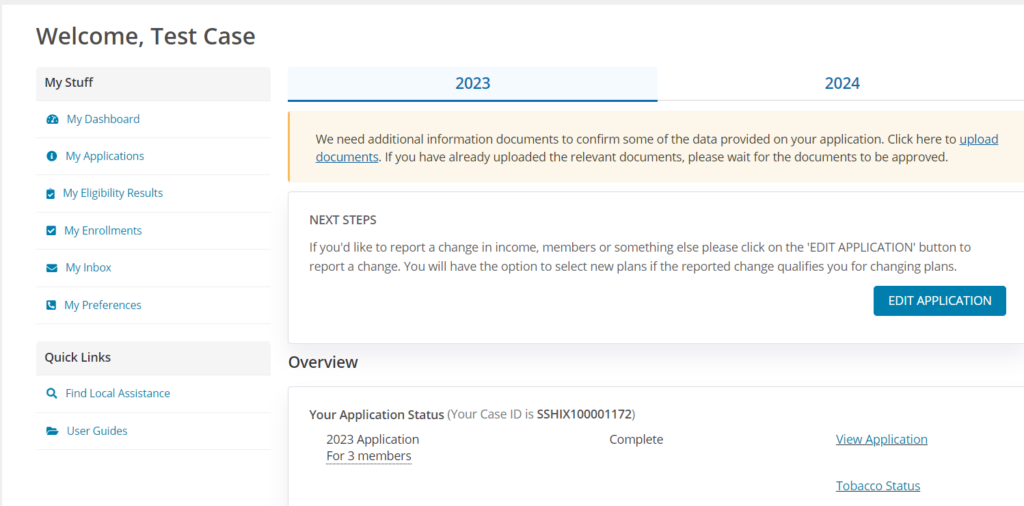In the top left corner of the image, there's a text stating "Welcome Test Case." Below it on the left side, a vertical menu of options is displayed, with section headings in black and individual options in blue. The first section is labelled "My Staff" and includes the following options: "My Dashboard," "My Applications," "My Eligibility Results," "My Environment," "My Inbox," and "My Preferences." Another section labelled "Quick Links" includes: "Find Local Assistant" and "User Guide."

On the right side, at the top, there are the years "2023" and "2024," with "2023" highlighted by a light blue background and an underline. Below this is a text box with a brown background that reads: "We need additional information/document to confirm some of the data provided on your application. Click here to upload documents. If you have already uploaded the relevant documents, please wait for the documents to be approved."

Further down, there's another text box under the heading "Next Steps." It explains: "If you would like to report a change in income, members, or something else, click the 'Edit Application' button below to report a change. You will have an option to select new plans if the reported change qualifies for changing plans." There is a blue button labeled "Edit Application."

At the bottom, it says "Overview" and "Your Application Status," followed by "Case ID." The status indicates "Three applications for three members complete." Below this, there are two blue buttons: "View Application" and "Tobacco Status."

This detailed caption aims to accurately describe the layout and content of the image.